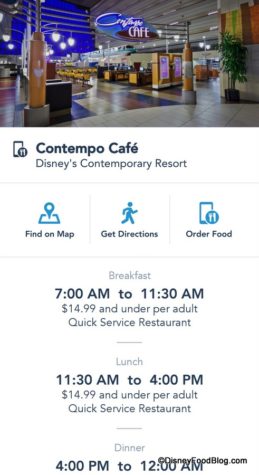The image features a screenshot set against a white background. At the top is a color photograph depicting the interior of a cafe, characterized by wood or wood-style flooring. Hanging from the ceiling, in neon-style lighting, an oval sign reads "Contempo Cafe." The scene shows numerous yellow chairs arranged in lines, although the image is slightly blurry.

Below the photograph, block text spells out "Contempo Cafe," followed by smaller blue text that reads "Disney's Contemporary Resort." Detailed information about meal timings and pricing is provided in organized sections:

- **Breakfast**: 7 a.m. to 11:30 a.m. – $14.99 and under per adult, designated as a quick-service restaurant.
- **Lunch**: 11:30 a.m. to 4 p.m. – $14.99 and under per adult, in bold blue text.
- **Dinner**: 4 p.m. to 12 a.m.

At the bottom right corner, a copyright icon is followed by the text "disneyfoodblog.com," indicating the source of the information.